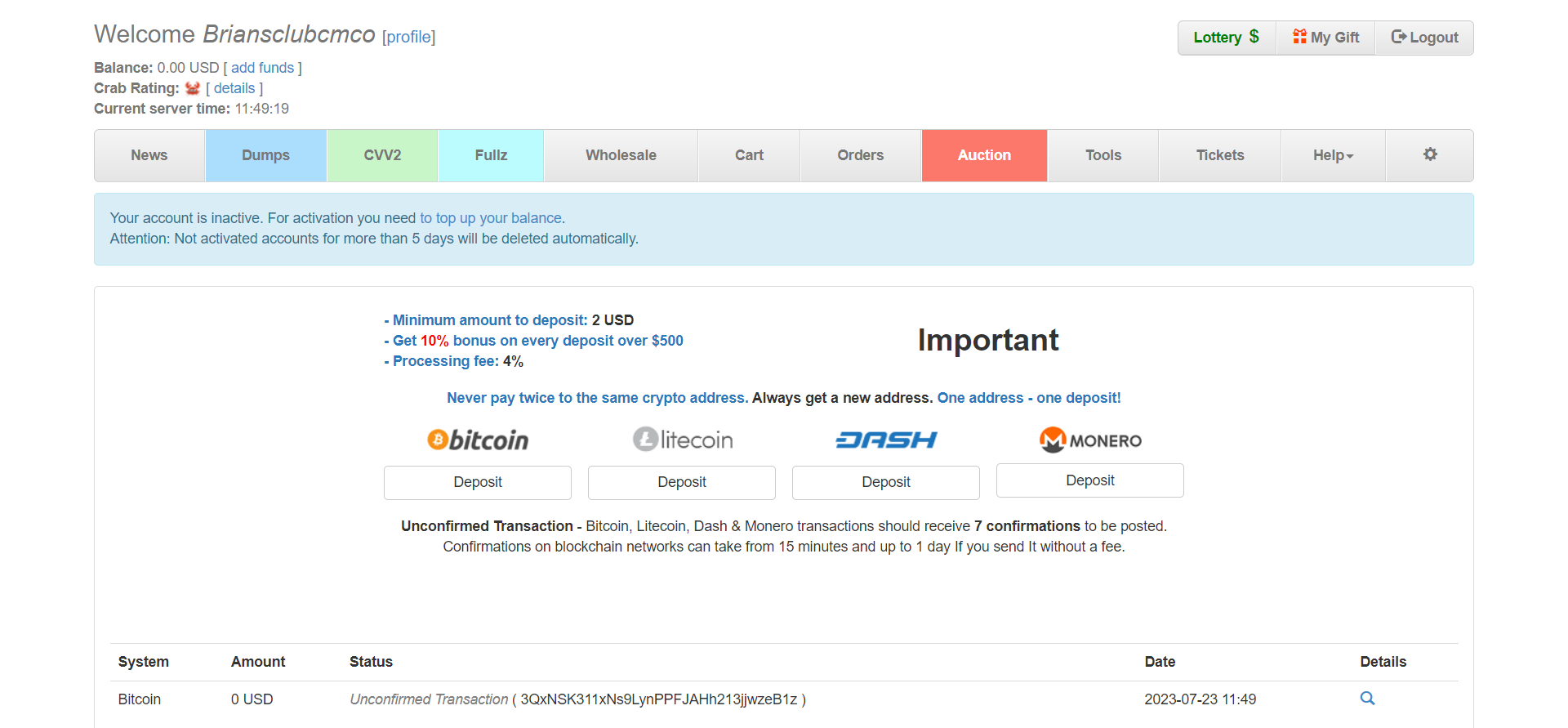Screenshot of a Webpage on a Computer Screen:

At the very top of the webpage, on the left-hand side, there is a welcome message followed by the user's name: "Welcome, Brian's Club." Below this, it shows "CMCO," the balance as "$0," and a blue button labeled "Add Funds." It also displays a "Crowd Rating" button next to which you can click on "Details." The current server time and a level indicator, "Level 4919," are also visible at the top.

On the right-hand side of the top section, there are three buttons: "Lottery" with a dollar sign, "My Gift," and "Log Out." Next to these, there's a navigation bar with multiple clickable items: "News," "Dogs," "CV," "V2," "FOLAs," "Wholesale," "Cart," "Orders," "Auction," "Tools," "Tickets," and "Help." The last icon in this bar is a small "Settings" icon.

Below the top navigation is a light blue banner with a warning on the left-hand side: "Your account is in NAFTA for activation. You need to top up your balance. Attention, not activated accounts for more than five days will be deleted automatically."

In the main body of the webpage, the following information is displayed:

- "Minimum amount to deposit: $2 US dollars."
- "Get 10% bonus on every deposit over $500."
- "Processing fee: 4%."

These tracts are written in blue text, except for "$2 US dollars" and "10% bonus."

To the right of this information, it states "Important" followed by: 
- "Never pay twice to the same crypto address" (in blue).
- "Always get a new address" (in black).
- "One address - one deposit!" (in blue text with an exclamation point).

Below this, there are cryptocurrency options for deposit:
- Bitcoin: a "Deposit" button.
- Litecoin: a "Deposit" button.
- Dash: a "Deposit" button in blue letters.
- Monero: a "Deposit" button.

An additional note states:

"Unconfirmed transaction: Bitcoin, Litecoin, Dash, and Monero transactions should receive seven confirmations to be posted. Confirmations on blockchain networks can take from 15 minutes up to one day if you send it without a fee."

At the very bottom of the screen, it shows a "System" status for a Bitcoin transaction:
- Amount: $0
- Status: Unconfirmed transaction
- A long transaction number

To the right, it shows the date and includes a "Search" button with the word "Details."